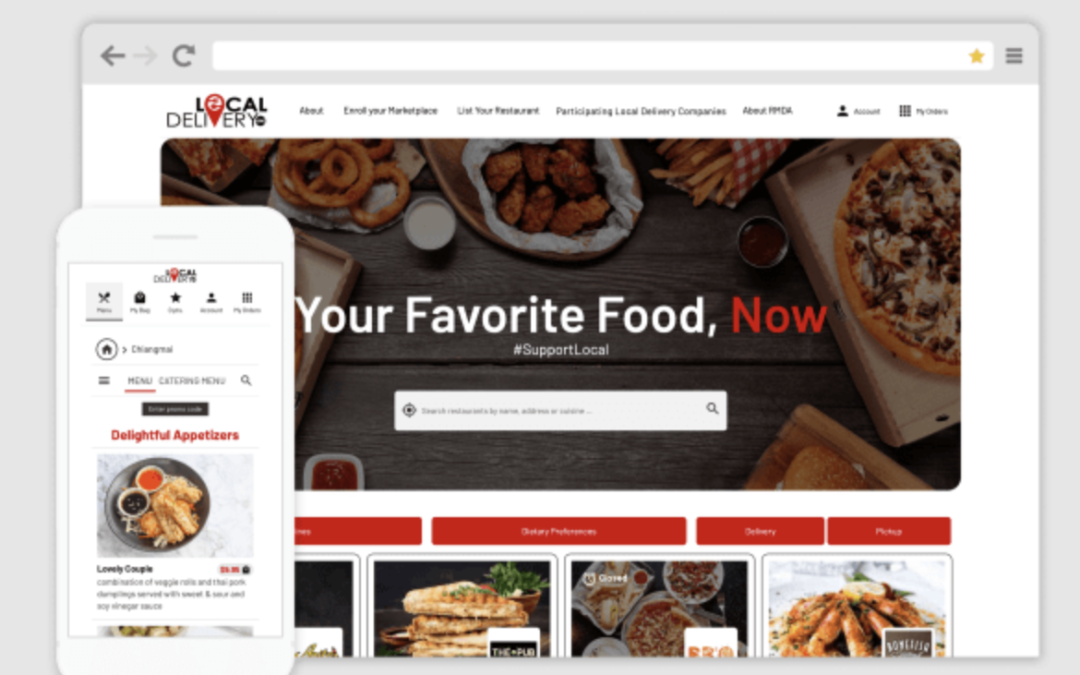This image showcases a website promoting local food delivery services, with a cleverly designed logo that integrates a red pin icon within the letters "L," "O," and "V" from "local" and "delivery." The website is presented both on a desktop screen and a mobile phone, illustrating its responsive design. 

On the desktop version, the central focus is a tempting array of food, featuring onion rings, chicken wings, French fries, pizza, and possibly chicken breast, alongside what seems to be either lobster or crab. A striking headline in the center reads "Your Favorite Food, Now," with "Now" highlighted in bold red text, while the rest of the phrase is in white. 

Below the headline is a search bar, inviting users to find their desired meals easily. The mobile version on the left displays the same theme, with text emphasizing "Delightful Appetizers" and a section titled "Lovely Couple." It suggests that users can explore further by clicking on various interface elements for additional information. The overall design is bright, engaging, and user-friendly, enticing viewers to explore the food delivery options available.